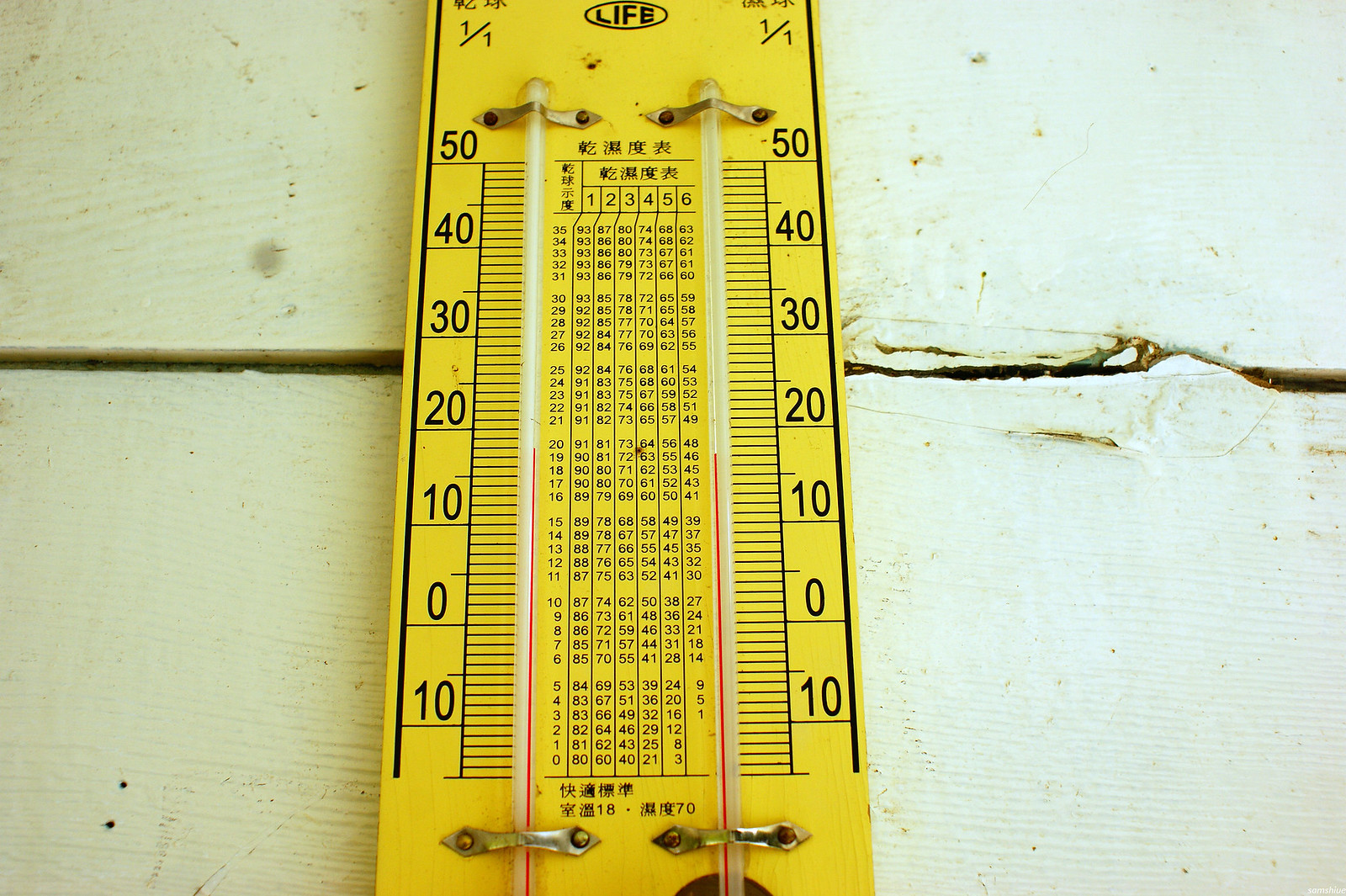This outdoor photograph showcases a vintage double thermometer mounted on a white clapboard wood wall. The wall's design features horizontal planks with visible gaps between them, and on the right side of the image, a knob and some brown marks are evident on the wood. The thermometer, elegantly crafted, consists of two glass mercury tubes, each displaying temperature measurements that start at 50 degrees and descend through 40, 30, 20, 10, 0, and then back up to 10 degrees. 

At the top of the thermometer, two horizontal rows of Asian characters are prominently displayed, accompanied by a vertical row of similar characters. Beneath this, the numbers one through six are neatly listed. Further down, multiple columns filled with numerous small numbers can be observed, though their specific significance remains unclear. The overall design and detailed markings contribute to the thermometer's intricate and enigmatic appearance.